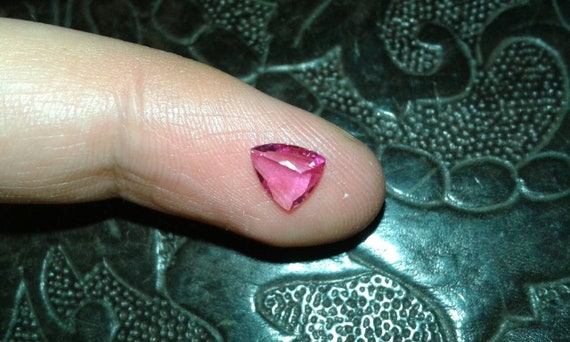In this close-up image, we see the tip of a light-skinned index finger, likely belonging to a Caucasian person, resting delicately on a glossy, blue-green patterned surface. The surface, reminiscent of a scaly texture with smooth areas, features multiple oval shapes and white-spotted patterns, almost looking like marble or the material of a purse. The focal point of the image is a small, shiny pink gemstone shaped like an inverted triangle or diamond, which is much smaller than the fingertip it's perched upon. The vibrant pink gem contrasts sharply against the intricate green backdrop, creating a striking visual composition.